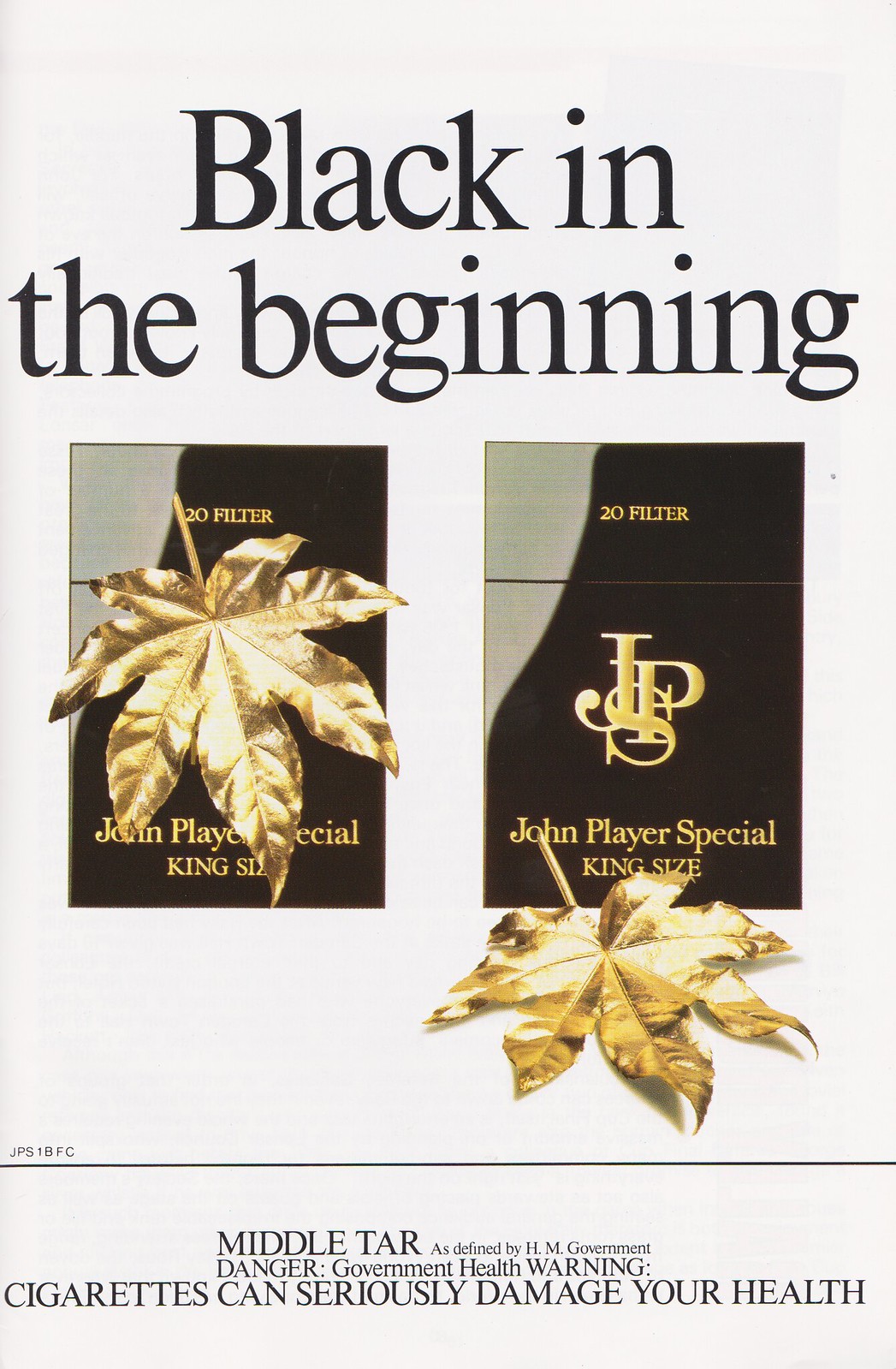This image is a rectangular, vintage cigarette advertisement poster, mostly featuring a tan off-white background. Dominating the top third of the image, there is bold black text split into two lines, reading "Black in the beginning." Centrally placed in the image are two identical packs of John Player Special King Size cigarettes. Each pack is predominantly black with a grayish curve in the upper left corner and adorned with gold details, including the text "20 filter" at the top, the intertwined initials "JPS" in the center, and the phrase "John Player Special King Size" at the bottom. Each pack is also paired with a golden tobacco leaf: one positioned in front of the left pack and the other lying on the table in front of the right pack. The bottom third of the image serves as a footer, demarcated by a horizontal pinstripe black line and containing a health warning. The warning, written in black print, states, "Middle Tar as defined by HM Government. Danger, government health warning. Cigarettes can seriously damage your health." The color palette prominently features off-white, black, gray, gold, yellow, and tan, contributing to the overall vintage and formal style of the advertisement.